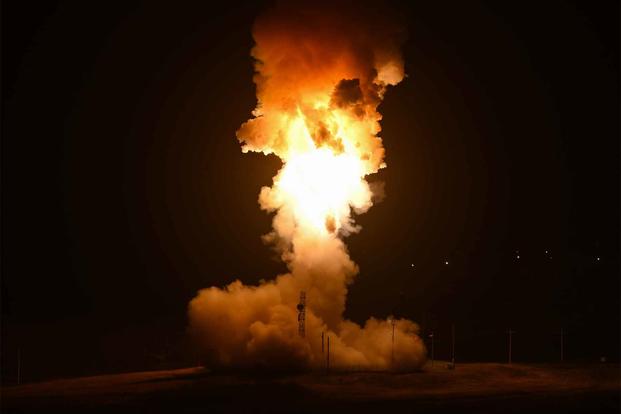The image depicts an intense, fiery scene that is either a rocket taking off or a large explosion, set against a completely dark, nighttime background. At the heart of the picture, a towering column of fire shoots straight up into the sky, with a large plume of smoke billowing around its base and rising upward. The fire is predominantly bright white at its core, transitioning through vibrant shades of yellow, red, and orange as it spreads outward, visibly lit from within by the searing heat. The ground below appears to be reddish-brown dirt or sand, possibly surrounded by fencing or related structures that could serve as guide towers for a rocket launch. To the right of the explosion, five white lights are arranged in pairs, hinting at distant buildings or towers across what seems to be a body of water, such as a river or lake, suggested by the distant lights flickering in the surrounding darkness.